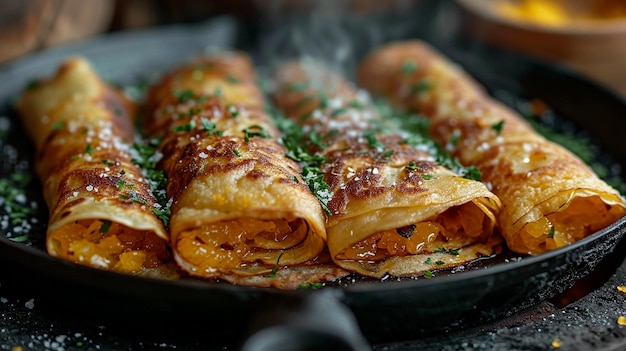A close-up shot captures a black platter adorned with four savory crepes. The centerpiece crepe, located at the middle left, is sharply in focus, showcasing its golden-brown texture. It is generously topped with finely chopped green onions or scallions, and visibly oozing with melted cheddar cheese. A light sprinkling of salt or Parmesan cheese enhances the savory presentation. The remaining three crepes, slightly blurred in the background, hint at similar fillings and toppings, maintaining the overall theme of cheesy delight intertwined with the fresh, zesty touch of green onions.